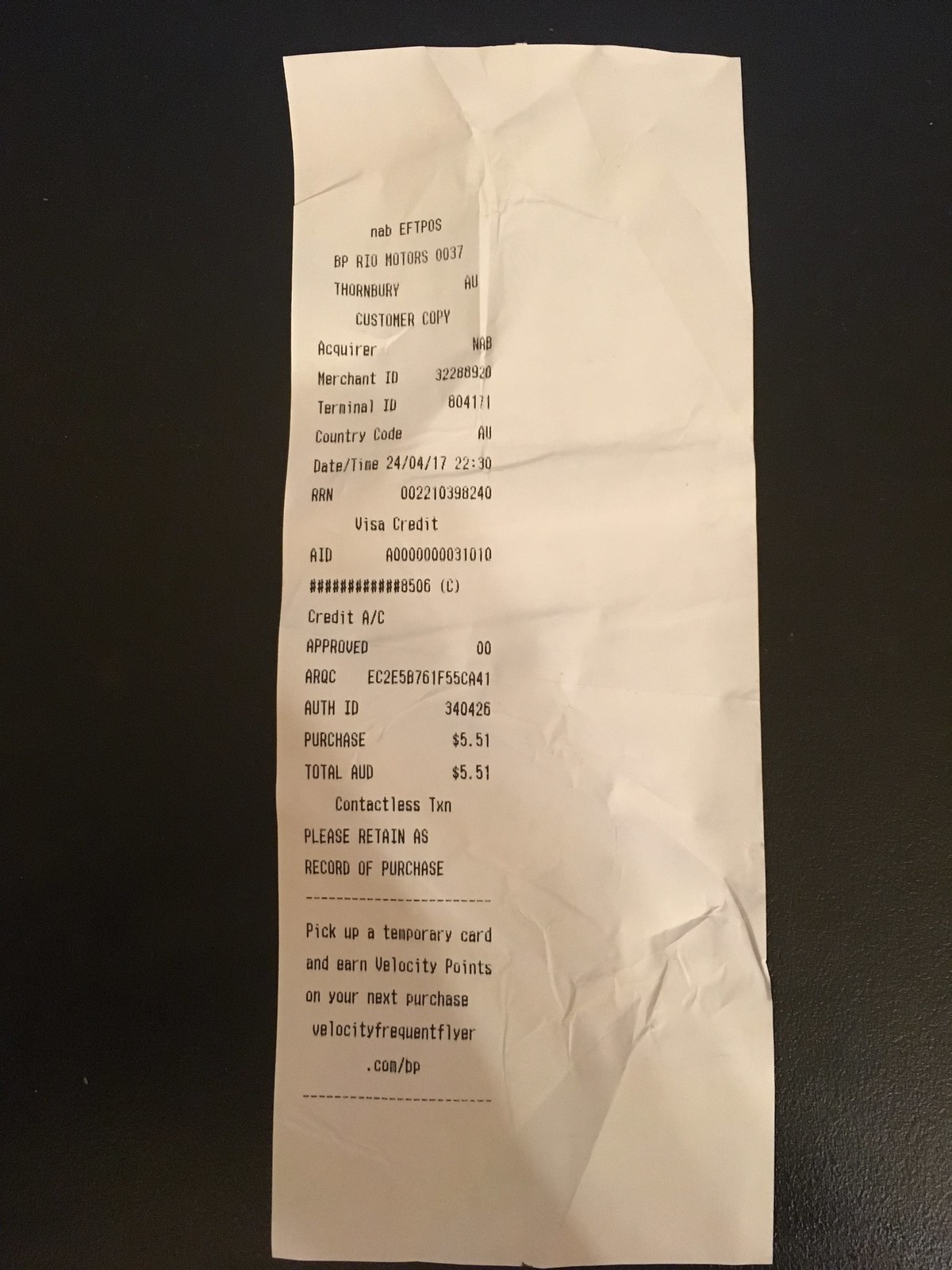**Descriptive Caption:**

A close-up photo of a white receipt resting against a black background reveals intricate details of a transaction. The header confusingly reads "NAB EFTPOS" followed by the line "BP RIO Motor 0037." Below it, the location is specified as "Thornberry BURY AU." The receipt is marked "Customer Copy" and identifies the "Acquirer" as "NAB." It includes respective IDs: "Merchant ID: 32288920" and "Terminal ID: 8041." The country is indicated by code "AU." The date and time are recorded as "24/04/17 22:30." Payment was processed as "Visa Credit" with the approval stamp "Credit A/C Approved." The total purchase amounts to $5.51, concluding with "Please retain as record of purchase."